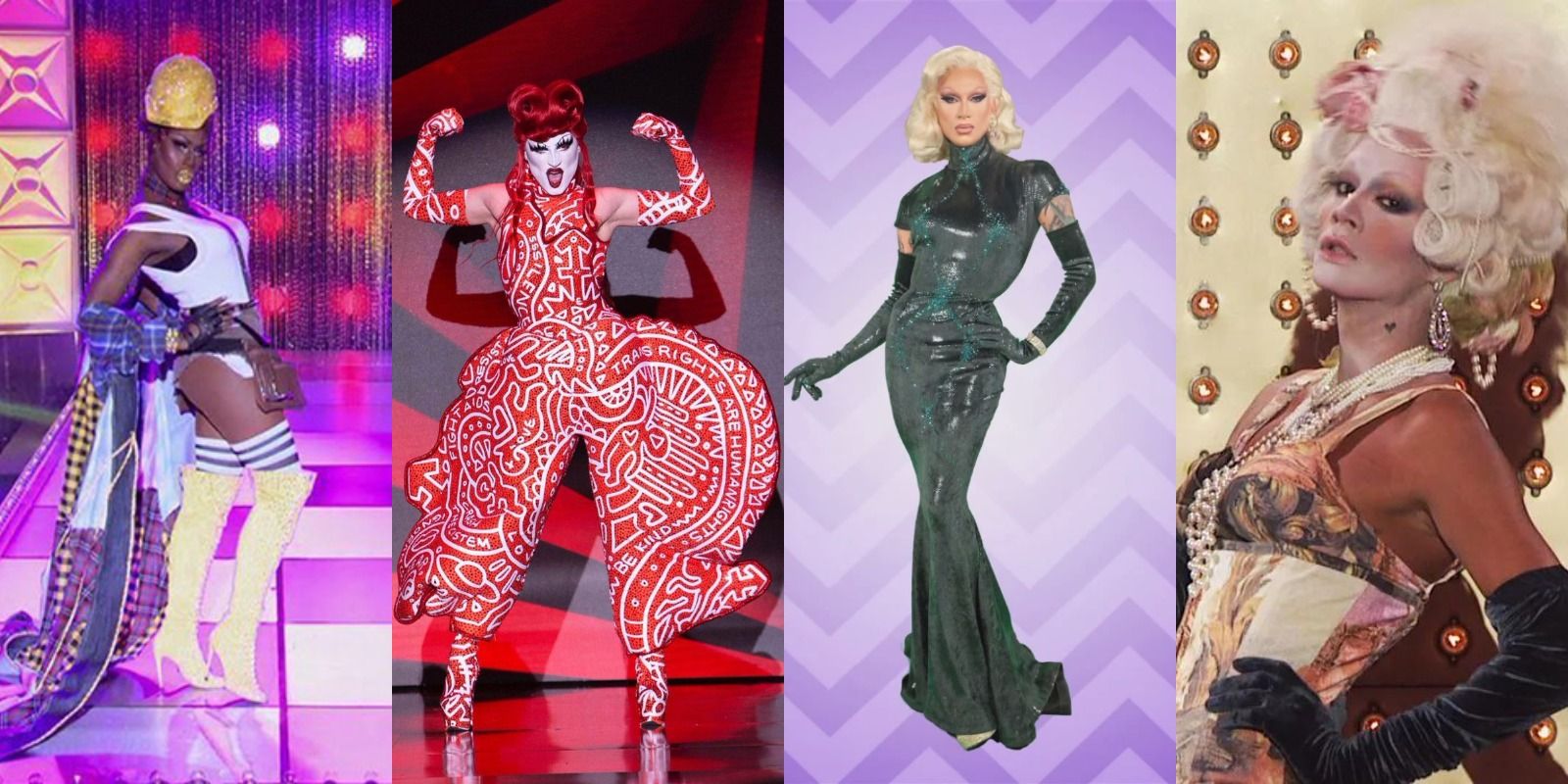The image is a horizontal collage comprising four vertical photos of celebrities or drag artists, each posing in elaborate costumes and heavy makeup against distinct colored backgrounds. On the leftmost side, against a purple stage with spotlights and a transparent curtain, stands a dark-skinned person with platinum blonde hair. They wear towering yellow high-heeled boots, a white outfit, and a decorative yellow hat, along with a bluish veil and cape-like scarves draping to the floor. The second image features a person against a predominantly red background, showcasing their muscles while donning a striking red and white Asian-inspired outfit with intricate patterns. This individual has vibrant red hair, a painted white face, and red boots. The third image captures an elegant figure with short blonde hair standing against a purple zigzag backdrop. They are dressed in a dark gray or greenish-gray gown with a sophisticated air. The final image shows another blonde individual leaning against an ivory wall adorned with gold details. They wear a white outfit, accentuated by long velvet gloves in a darker shade. The collective styling emphasizes high fashion and theatrical flair.